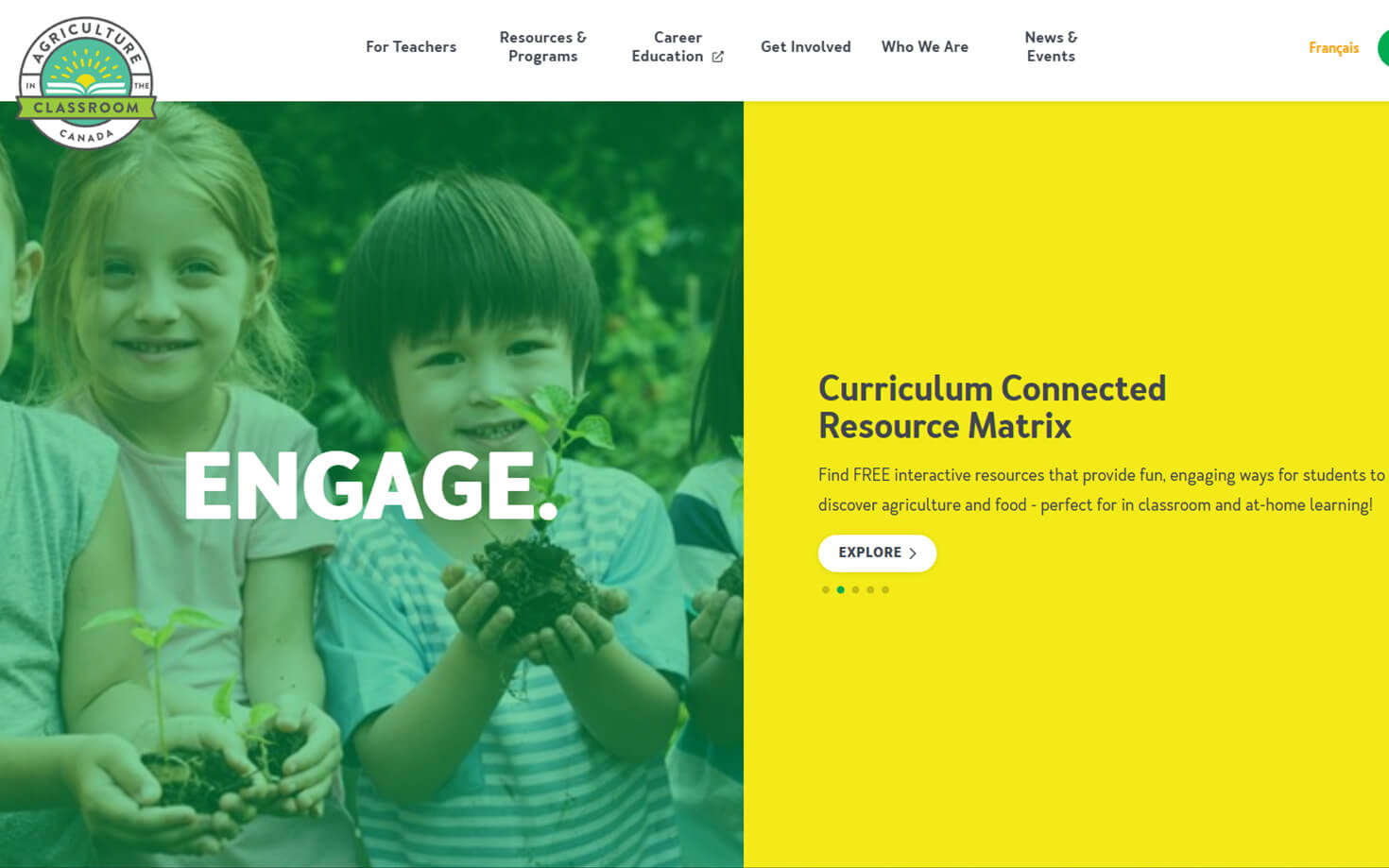This image is a screenshot taken from a computer screen, featuring the homepage of an agriculture education website in Canada. At the top, within a circular emblem, the words "Agriculture Classroom" are prominently displayed, with "Classroom" highlighted on a green banner. Adjacent to this emblem are navigational links in black print: "For Teachers," "Resources and Programs," "Career Education," "Get Involved," "Who We Are," and "News and Events."

In the main section of the image, there is a photograph depicting four young children, though only two are fully visible while the others are partially obscured, showing only their hands or a glimpse of their hair. The children are engaged in an activity, holding a plant with exposed soil and roots, suggesting an educational hands-on experience in agriculture.

On the right side of the screen, there is a yellow square containing the text "Curriculum Connected Resource Matrix," accompanied by an "Explore" button that encourages users to learn more.